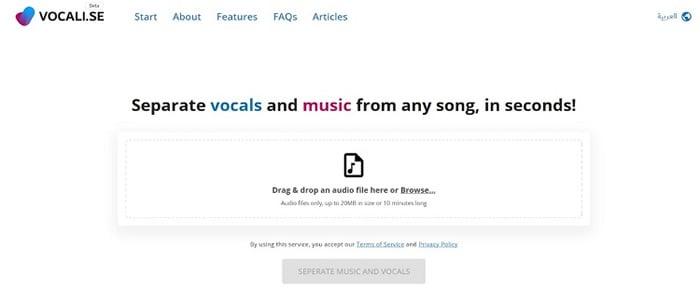On this webpage, presented against a white background, black and dark-colored text predominates with some sections highlighted in burgundy and navy blue. In the upper left corner, there is a blue and purple logo with the text "Vocalize" spelled out as "V-O-C-A-L-I dot S-E" accompanied by a "Beta" label above it. To the right of the logo, there are navigation buttons labeled Start, About, Features, FAQs, and Articles sequentially, ending with a globe icon on the far right. 

Centrally positioned on the page, bold text proclaims, "Separate vocals and music from any song, in seconds!" with the word "vocals" in blue and "music" in burgundy. Below this headline, a rectangular box invites users to "drag and drop an audio file here or browse…" with instructions indicating that files should be up to 20 megabytes in size or 10 minutes long. Although the text appears slightly blurred due to low resolution, these details are discernible.

Further down, a notice states that by using the service, users accept the terms and services and privacy policy. At the bottom, a gray button labeled "Separate music and vocals" remains inactive until an audio file is uploaded.